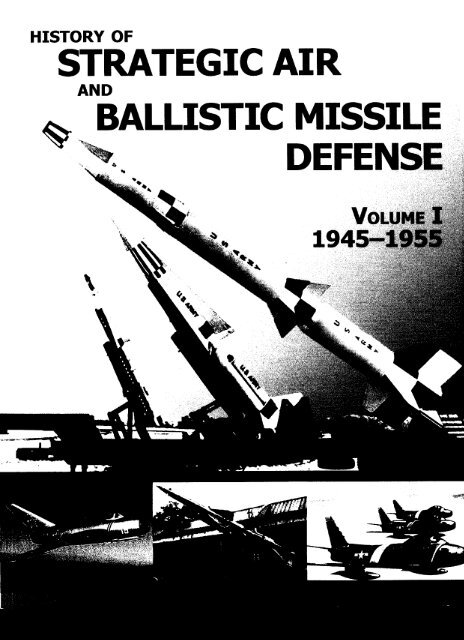The image, likely the cover of a textbook titled "History of Strategic Air and Ballistic Missile Defense," Volume 1, 1945-1955, showcases various elements related to missile and air defense between the end of World War II and the start of the Vietnam era. Rendered in black and white, it prominently features three U.S. Army ballistic missiles pointed skyward with a distinctive black and white checkered pattern three-quarters up their length. The cover also includes several aircraft, with three fighter jets visually clustered in the bottom right corner, one additional fighter jet at the bottom left, and what seems to be a missile silo in the bottom middle section. Unfortunately, the shadows from photocopying obscure some details, rendering parts of the image dark and challenging to interpret.